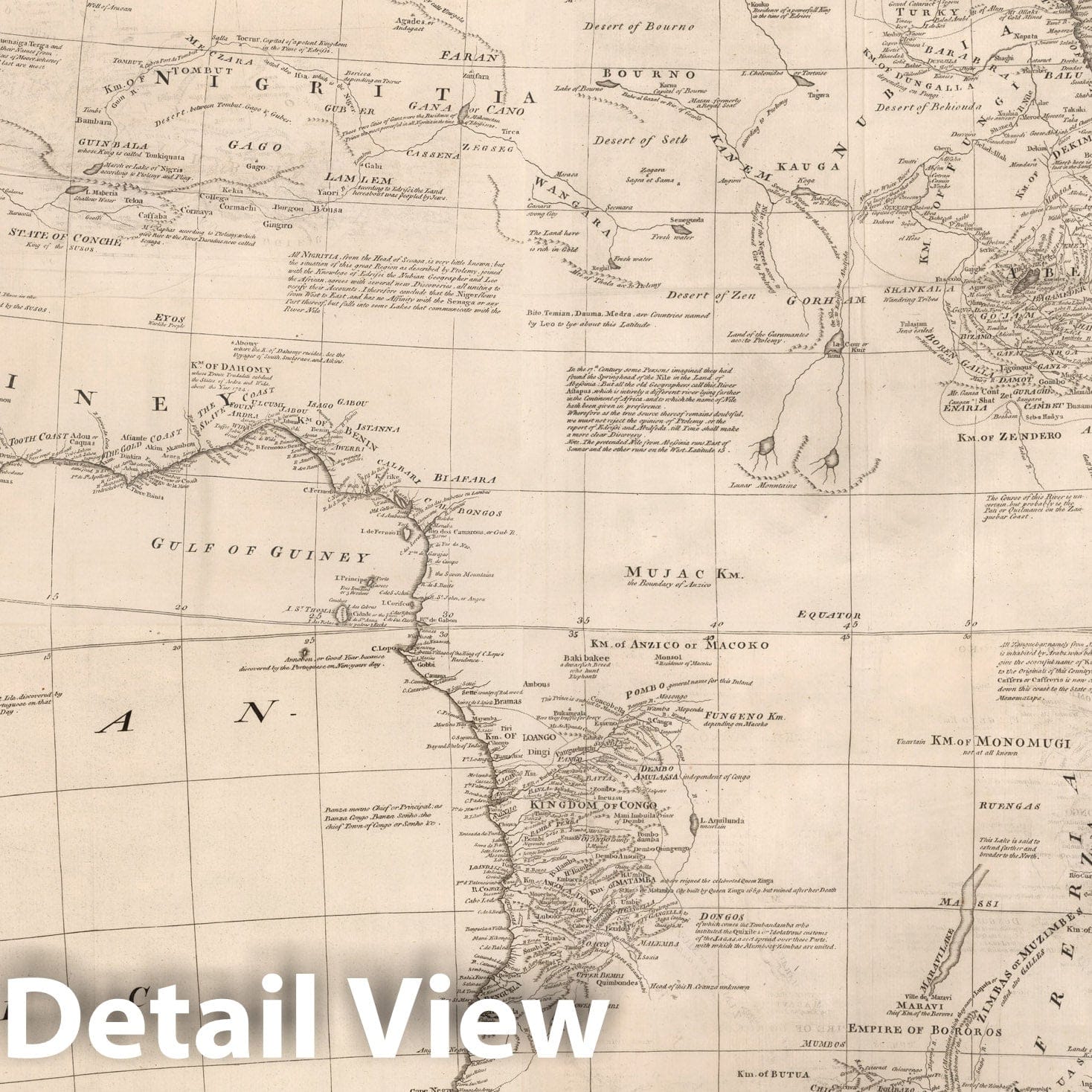This detailed image features an old hand-drawn map, possibly dating back to the 1700s or early 1800s, drawn on beige parchment paper. The bottom left corner of the map showcases a coastline labeled "Gulf of Guinea," suggesting it depicts part of the African continent. Overlapping this map in the same bottom left corner is white text with a gray drop shadow reading "Detail View." At the top left, the map is marked "Negritia," though the exact placement and spelling of regions can be unclear due to the antiquated nature of the map and the often small and difficult-to-read black text scattered across the image. Distinct locations include "Kingdom of Congo" at the bottom and "Empire of Bororos" on the bottom right.